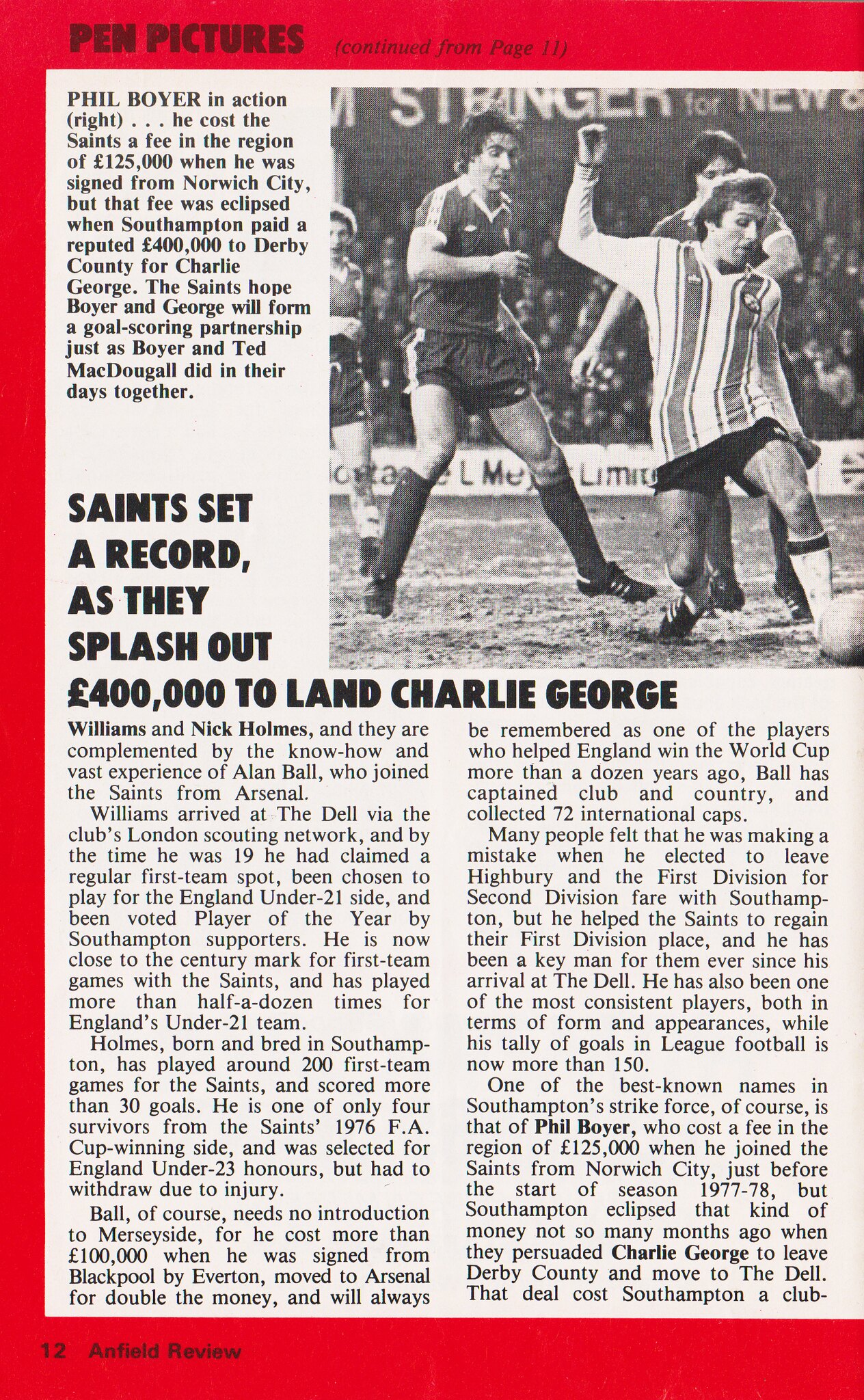The image depicts a magazine clipping encased by a red border on three sides, with prominent text at the top stating "Pen Pictures" and noting the continuation from page 11. The main article, headlined "Phil Boyer in action," details how Phil Boyer was acquired by the Saints for approximately £125,000 from Norwich City, a cost that pales in comparison to the £400,000 Southampton paid Derby County for Charlie George. The Saints hope to see Boyer and George form a successful goal-scoring partnership akin to the one Boyer had with Ted McDougal. To the right of the text, there is a black-and-white photograph featuring four soccer players in action. The article spans two columns and includes a subtitle: "Saints set a record as they splash out £400,000 to land Charlie George." At the bottom left corner, the page is numbered 12, indicating it is part of the "Ant Field Review."